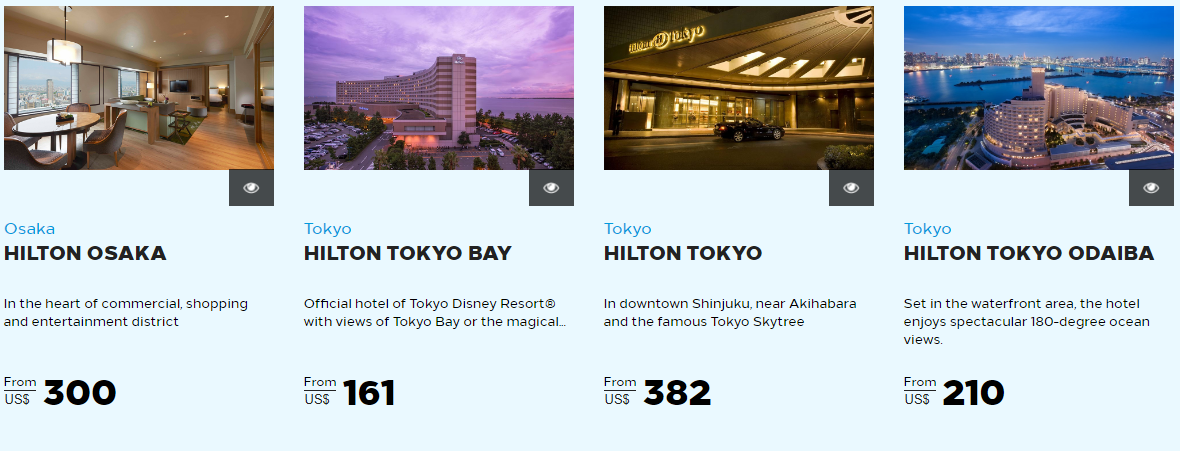Detailed Caption: 

The image showcases four columns featuring different hotel destinations in Japan, primarily from the Hilton chain, each with detailed information and images. 

1. **Hilton Osaka**: Located in the heart of Osaka's bustling commercial, shopping, and entertainment district, this hotel offers convenience and luxury with room rates starting at USD $300. The image depicts a luxurious hotel interior, highlighting a spacious and elegant design.

2. **Hilton Tokyo Bay**: Official hotel of the Tokyo Disney Resort, this location offers enchanting views of Tokyo Bay. Rooms are priced from USD $161. The partial image showcases a view suggestive of its magical ambiance, fitting for its proximity to the famed resort.

3. **Hilton Tokyo**: Situated in downtown Shinjuku, near Akihabara and the iconic Tokyo Skytree, this hotel provides a central location for exploring Tokyo. Room prices begin at USD $382. The image displays a detailed hotel interior, capturing the blend of modernity and comfort.

4. **Hilton Tokyo Odaiba**: Set in the Odaiba waterfront area, the hotel boasts stunning 180-degree ocean views, with room rates starting at USD $210. The image features the hotel's exterior as viewed from a distance, emphasizing its prime waterfront location and scenic surroundings.